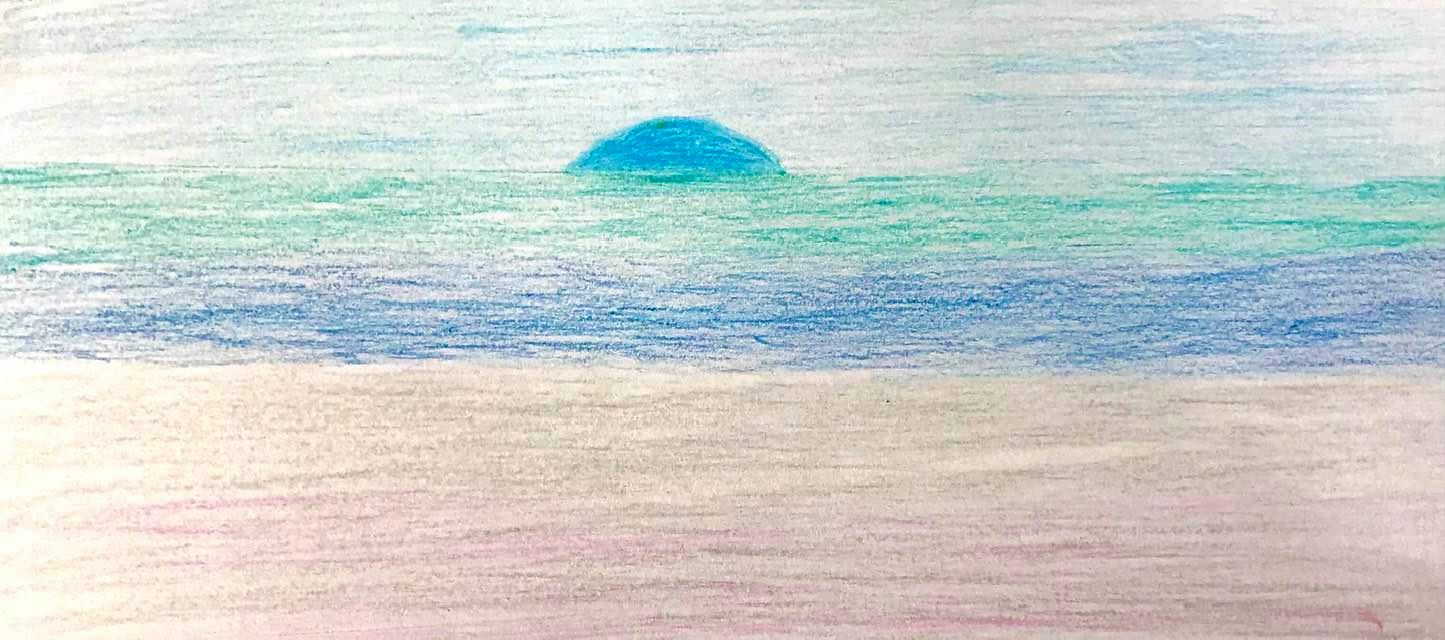This artwork, seemingly created with colored pencils on white paper, exhibits a minimalist beach scene rendered in horizontal strokes. At the base of the composition, a reddish-brown band suggests the sandy shore, smoothly transitioning to lighter tan and gray shades as it extends upward. This sandy expanse is bordered by a darker blue swath, indicating the immediate shoreline, while a lighter turquoise hue represents the distant ocean. 

Above this aquatic expanse, a subtle darker blue sky emerges, softly shaded to convey a delicate atmospheric effect. Central to this scene is a prominent, darker blue half-circle, which could be interpreted as a wave or an island positioned against the horizon. The artwork is characterized by its simplicity, with most of the colors appearing lightly applied, giving an airy, almost ethereal quality to the scene. Notably, the teal half-circle stands out with a more concentrated and fluorescent intensity, drawing the viewer’s focus amidst the otherwise gentle, muted palette.